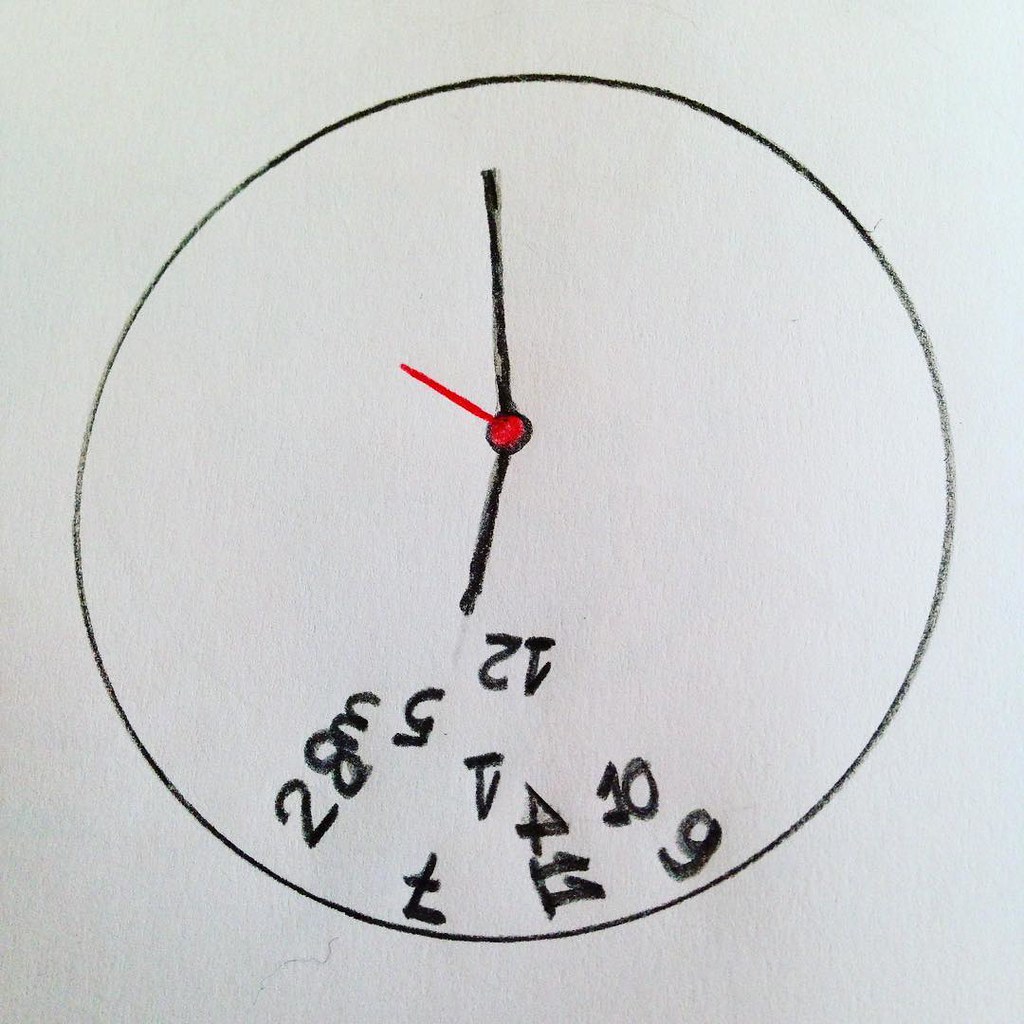This is a child’s drawing of a clock on a piece of white paper. The circle, likely traced using a bowl and drawn with a black charcoal pencil or crayon, contains clock hands indicating a time close to 6:58 and 50 seconds. The clock's hour and minute hands are black, while the second hand is red and slightly off-center towards the top of the circle. At the bottom of the clock face, there is a jumbled collection of numbers that were supposed to be around the clock. The numbers include an upside-down 12 and 1, a backward 3 and 5, an upside-down 7, a sideways 4, an angled 9, and 10, with 11 written to the right. Additionally, there are a 2 and 8 next to the circle, creating a disorganized spread of numbers, which might suggest the drawing is intended to assess cognitive efficiency.